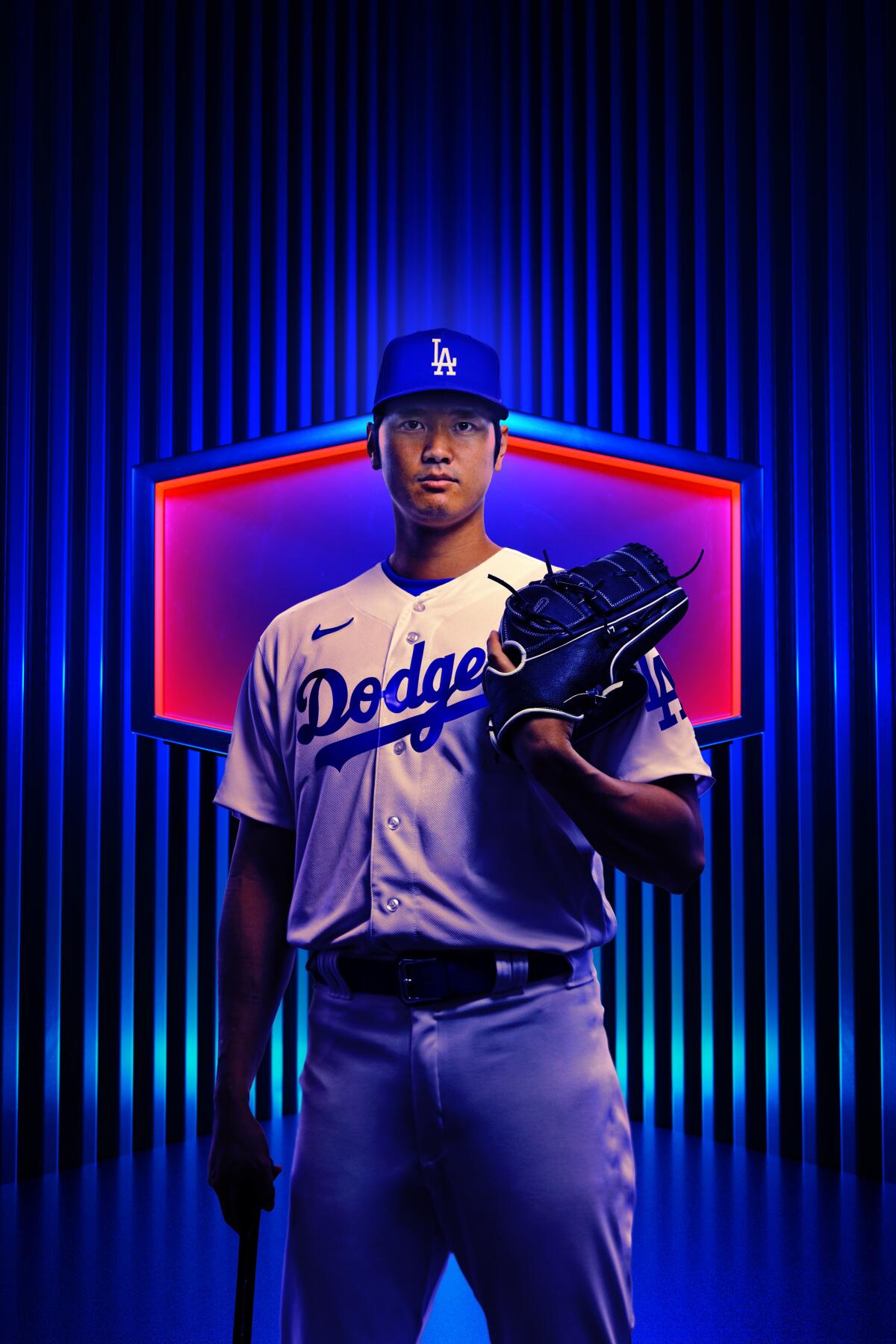In this vertically oriented rectangular image, we see an advertisement-like photograph featuring a Los Angeles Dodgers baseball player. The player is standing face forward, captured from the knees up. He is dressed in the iconic white Dodgers uniform with blue lettering, and he wears a matching blue baseball cap. His left hand is holding a baseball glove, which is curled upward against his chest.

The background is a striking composition of blue neon strips that run vertically from the bottom of the image to the top, set against a black backdrop. Directly behind the player's shoulders and head, there is an octagon-shaped neon light in red and blue, adding an eye-catching halo effect that further accentuates the player's figure. The overall effect is dynamic and dramatic, perfectly suited for a high-impact advertisement.